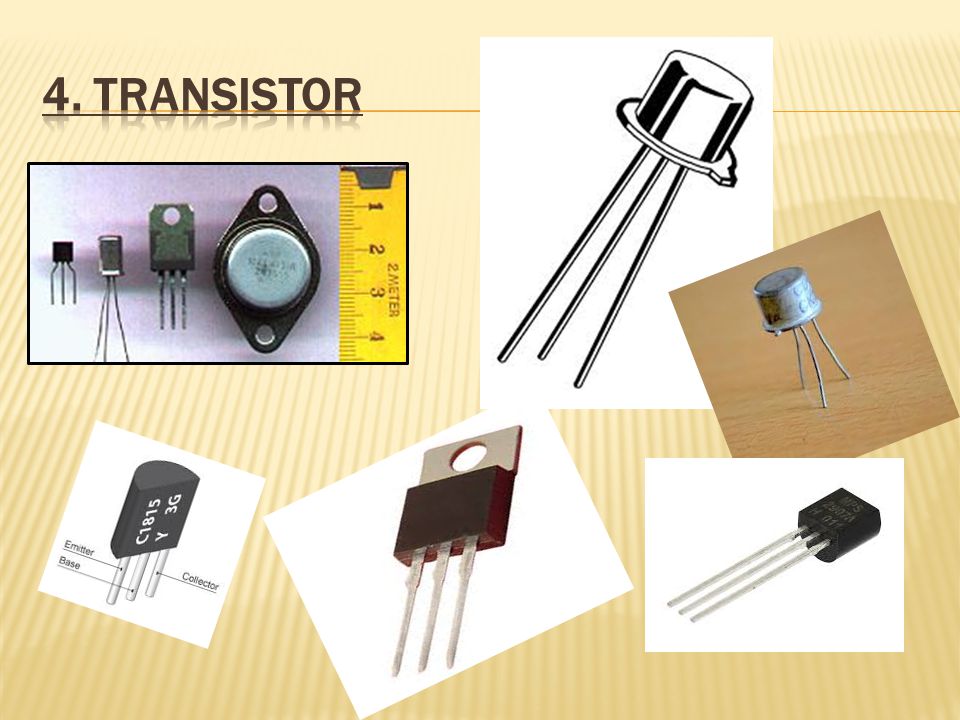At the top of the slide, the title reads "For Transistors." The slide contains various images depicting different types of transistors. Each transistor features three spiky legs, resembling pins, and they are presented in different cases. One set of images displays a clipart version of a transistor where these spiky legs are connected to an object shaped like a thimble. Another arrangement shows the spiky legs attached to a rectangular, dark-colored box.

Additionally, there is an image showing a transistor next to a yellow ruler for scale. This part of the slide includes four separate images, highlighting various perspectives and details of the transistor’s structure. The detailed depiction allows for a clear understanding of the transistor’s physical configuration and size relative to the ruler.